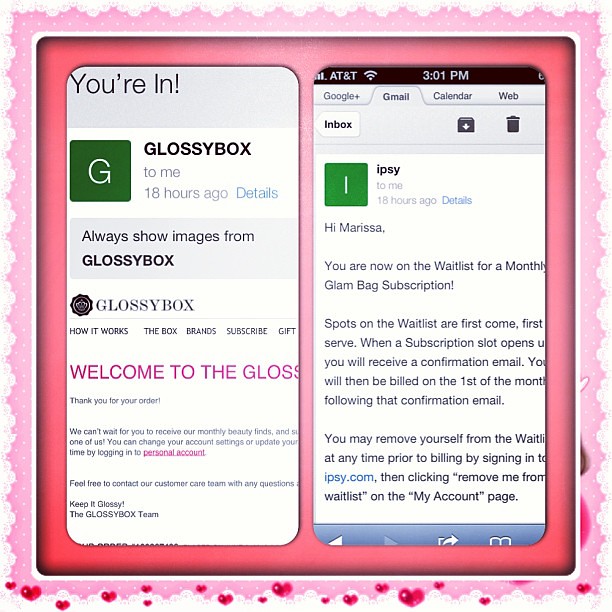The image features two side-by-side screenshots from a phone, each framed within a light pink border adorned with small, darker pink hearts at the bottom. Both screenshots are set against a pink background. The left screenshot shows an email from Glossybox, identifiable by a green square with the letter 'G' at the top. The email reads: "You're in! Welcome to the Glossybox. Thank you for your order. We can't wait for you to receive our monthly beauty finds. You can change your account settings or update your timing by logging into your personal account. Feel free to contact our customer care team with any questions. Keep it glossy, The Glossybox Team." Some text appears to be cut off. The right screenshot displays the AT&T logo at the top left corner with a time stamp of 3:01 PM, and highlights a Gmail tab within the Inbox. This email is from Ipsy, addressing a person named Marissa: "Hi Marissa, you are now on the waitlist for a monthly Glam Bag subscription. Spots on the waitlist are First Come, First Serve. When a subscription opens up, you will receive a confirmation email and will be billed on the first of the month following that. You may remove yourself from the waitlist at any time by signing into ipsy.com and clicking 'remove me from the waitlist' on your account page."